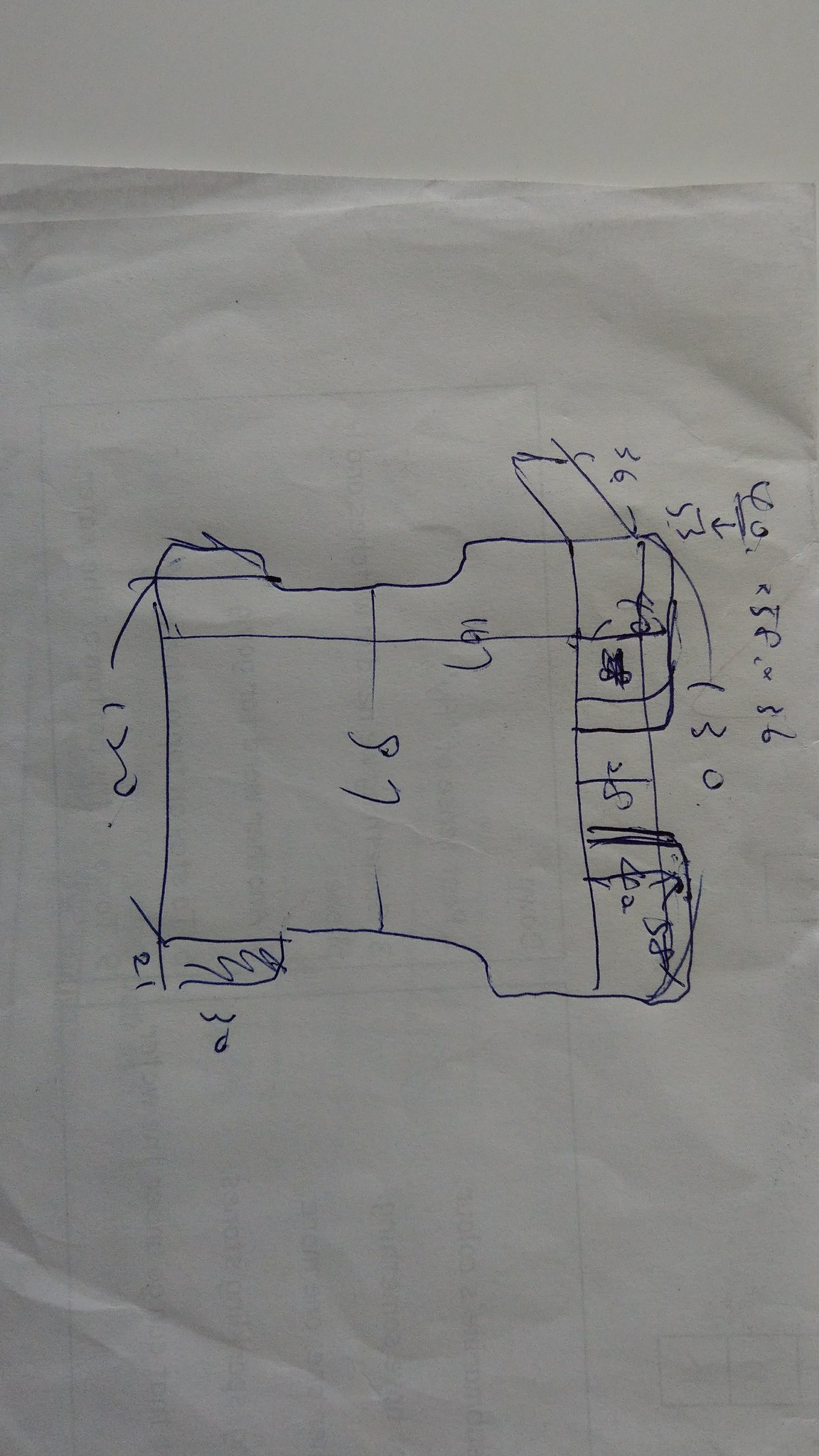This portrait-style image, significantly longer than it is wide, captures a crinkled white piece of paper featuring intricate pen drawings. Dominantly depicted is a puzzle-like shape, carefully outlined in pen, with various additional markings and sections that add depth to the design. 

In the bottom left corner, a rectangle is prominently filled with dark scribbles, contrasting sharply with another rectangular area in the top left corner that remains unfilled, allowing the white of the paper to show through. Stretching across the middle of the puzzle-shaped figure are two straight horizontal lines, providing a sense of alignment and structure. 

Approximately an inch from the top of this puzzle figure, a horizontal line extends from the left edge to the right, while another straight vertical line runs perpendicularly from near the top of the figure down to the bottom, about an inch from the right edge of the puzzle. 

Adjacent to these lines, particularly on the right side of the paper, are several scribble marks distributed inside and surrounding the rectangular shapes in the top-right corner of the puzzle form. Additionally, scattered random numbers are present, rotated 90 degrees clockwise, necessitating a head tilt to the right in order to read them correctly. This combination of elements creates a complex and visually engaging piece that piques curiosity and encourages closer examination.